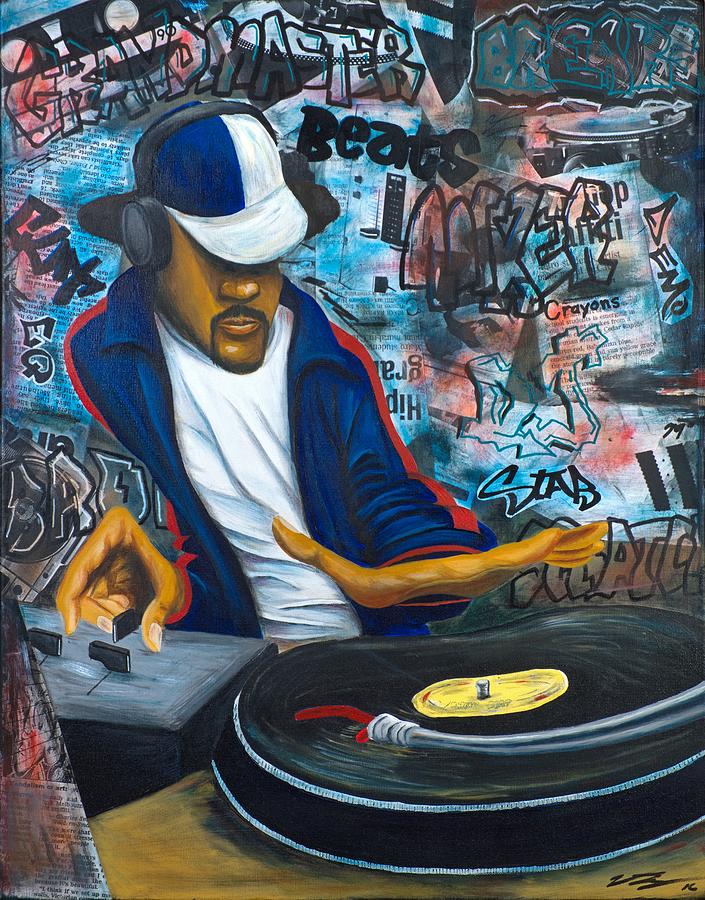This detailed artwork, resembling a caricature or cartoonish graffiti, depicts an African American DJ, characterized by his attire and the equipment he is using. He wears a blue track jacket with red stripes down the shoulders, a white and blue baseball cap, and a white t-shirt. His cap is distinctively split in color—one half blue and the other white, with a white bill. He also dons headphones, and his eyes are obscured by the cap, though his mustache and Fu Manchu chin hair are visible. The DJ is engaged with two turntables, poised to spin records, which exemplifies his role in the music scene.

The background is an intricate collage of graffiti with multiple words, including "Grandmaster," "Beats," "Stab," "Crayons," and "Nike." These words are set against a backdrop that mimics a newsprint in a bluish hue, adding layers of complexity to the image. Additionally, the letters "D-E-M" are visible on the right side. The bottom right corner features a subtle signature alongside the number "16," likely denoting the artist or specific artwork details. This mural, embodying the vibrant spirit of urban street art, possibly adorns a wall, emphasizing the cultural significance of the DJ within this animated and expressive context.